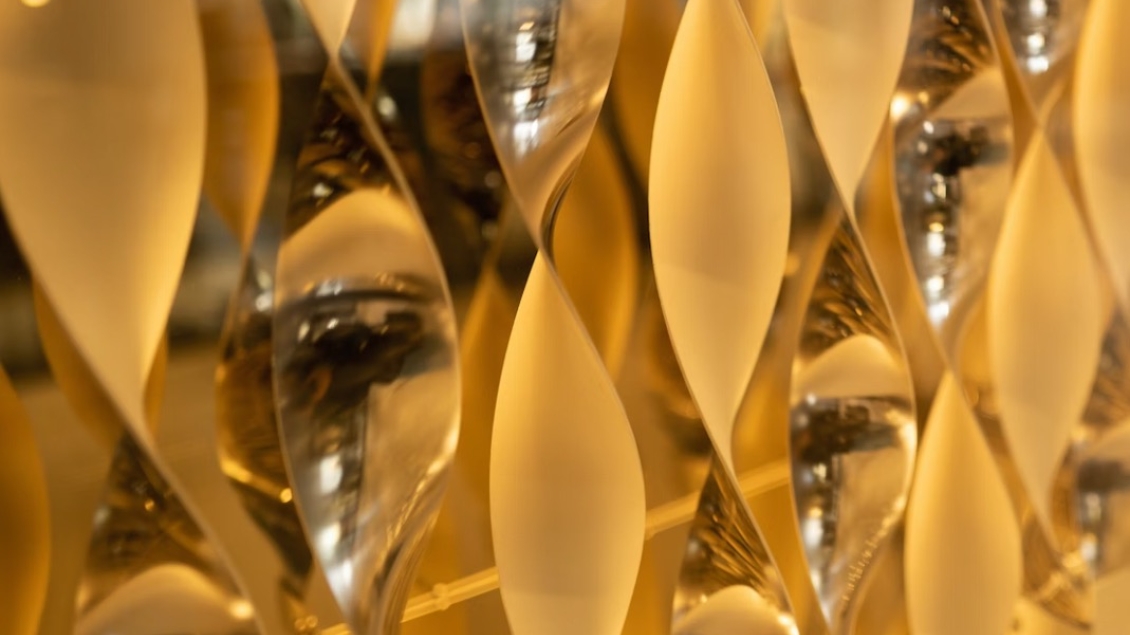The image is a horizontally rectangular, close-up photograph of twisted party decorations, possibly streamers or fringes, with no discernible background or border. The decorations consist of a twisted pattern predominantly in shades of creams, yellows, and silver. The silver portions are highly reflective, resembling droplets of water or a mirror-like surface, contrasting with the non-reflective, creamy yellow bands. These twisted decorations are aligned next to each other in a line, with approximately seven or eight of them visible. The image is brightly lit, providing clear visibility of the details and vivid colors of the decorations.